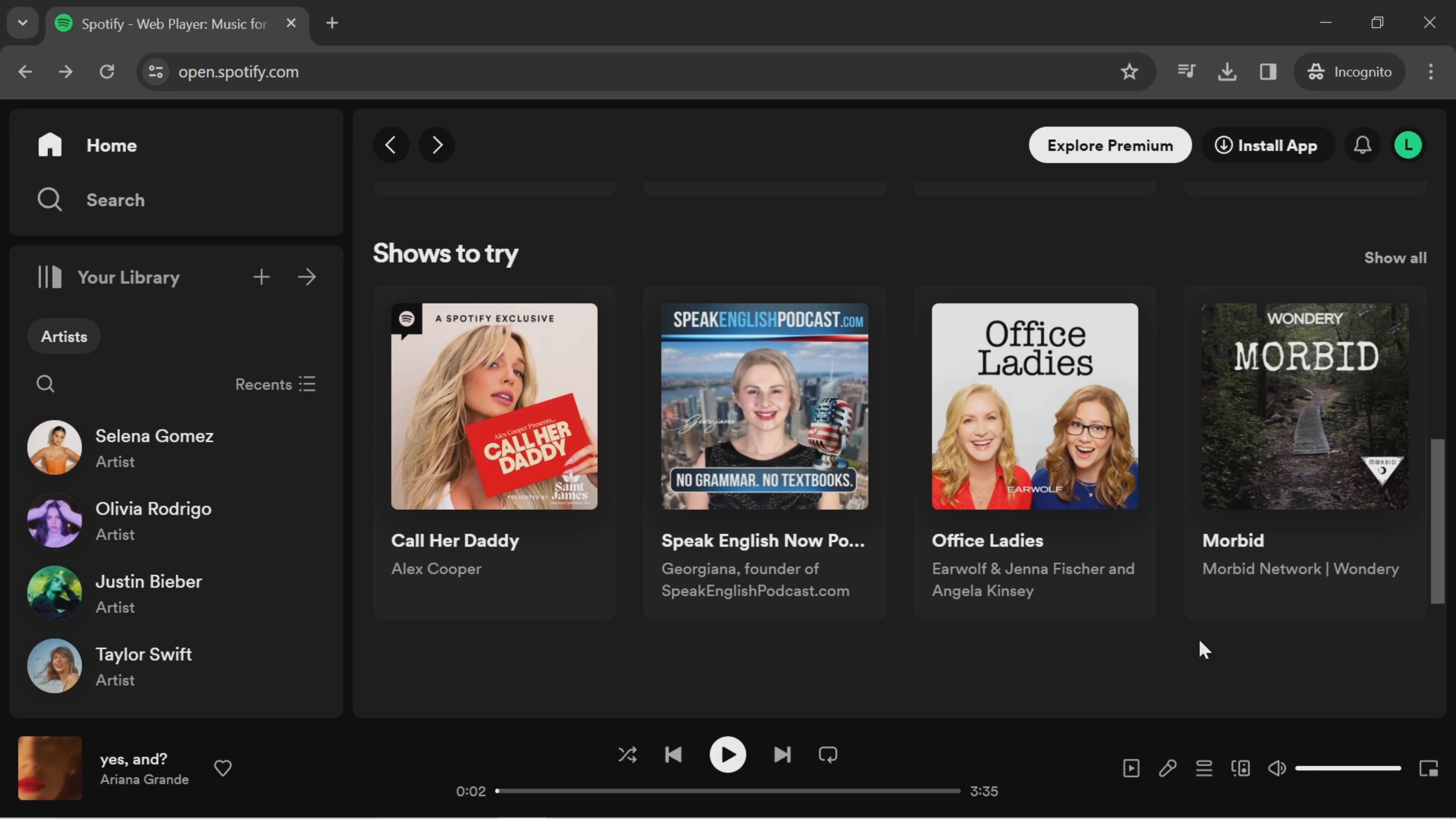The image is a detailed screenshot of the Spotify Web Player, captured using the Google Chrome browser in Incognito mode. The browser's interface features the recognizable Google Chrome logo at the top, along with the open.spotify.com URL in the address bar. To the left of the URL bar, navigation icons for 'back,' 'forward,' and 'refresh' are visible. To the right of the URL bar, there are icons for a 'music note,' 'download,' and an indication that the browser is in Incognito mode. 

On the Spotify interface, the sidebar menu lists options: 'Home,' 'Search,' 'Your Library,' and 'Artists,' with specific artists such as Selena Gomez, Olivia Rodrigo, Justin Bieber, and Taylor Swift mentioned. On the right side of the interface, there's an option to 'Explore Premiums,' and a clickable button to 'Install App,' accompanied by a notification bell.

Further down, there's a section featuring four podcast titles, each with its own thumbnail. From left to right, the podcasts are listed as "Call Her Daddy," "Speak English," "New Podcasts," "Office Ladies," and "Morbid."